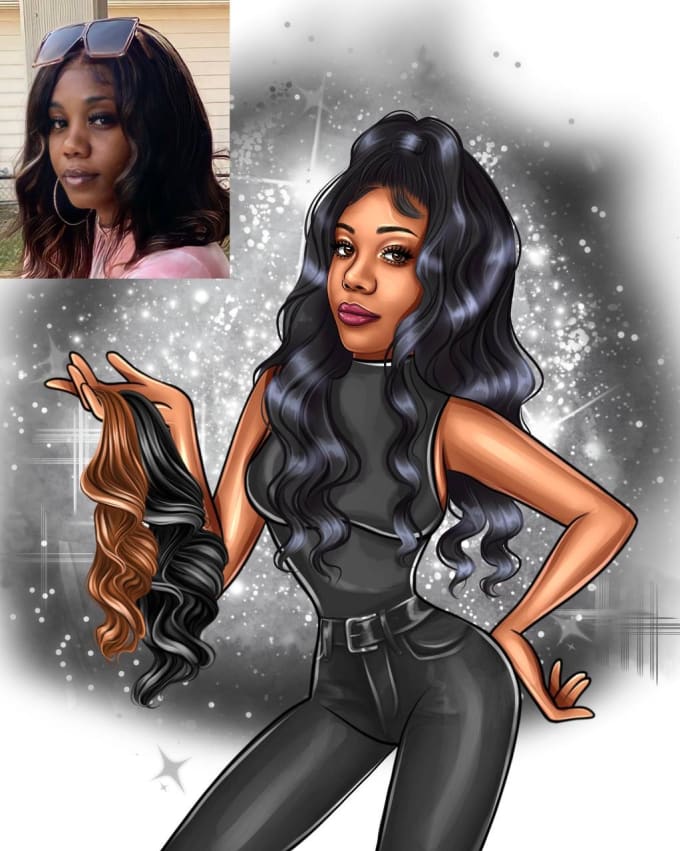The image showcases both a real photograph and a cartoon caricature of a black woman. The photograph, located in the upper left corner, depicts the woman with brown, shoulder-length hair, a pink top, and large sunglasses positioned on her head. She is sporting a loop-style earring and dark lipstick, posing against a light yellow wall with visible grass and a fence behind her.

The predominant part of the image, about 75-80%, features a detailed cartoon version of the same woman. In this animated depiction, she is shown with much longer, waist-length black hair and dressed in a tight-fitting, sleeveless black shirt, black pants, and a black belt. Her left hand rests on her hip, while her right hand is raised palm-up, holding two hair extensions—one brown and one black. The background of the cartoon is vibrant and sparkly, filled with white and gray star shapes and circles, adding a dynamic contrast to the stillness of the photograph in the upper left.